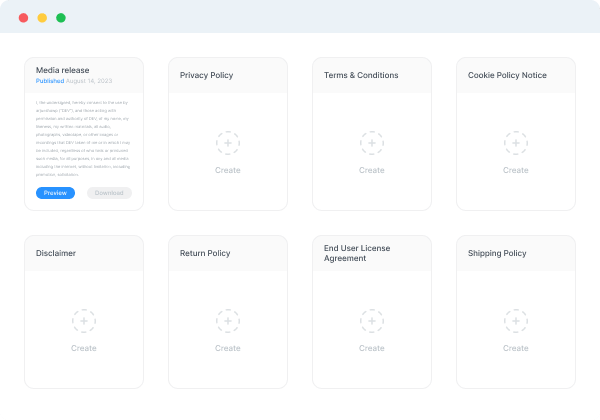The image depicts a somewhat cluttered interface, possibly related to content management or website administration. The upper left corner of the image is predominantly white, containing three small, aligned dots: one red, one yellow, and one green, reminiscent of window control buttons found on MacOS applications.

Below this section, the layout consists of eight distinct boxes arranged in two rows of four. The detailed descriptions of the boxes are as follows:

1. **Media Release**: This box has "Media Release" prominently displayed in bold black text. Beneath it, "Published" is written in blue, and a date, "August 14th, 2023," is noted in light gray. Further below, there are two buttons – a blue one labeled "Preview" and a grayed-out one labeled "Download."
2. **Privacy Policy**: This box features a dotted circle containing the word "Create" with a plus sign in the middle. The word "Create" is also displayed beneath the circle.
3. **Terms and Conditions**: This box is dedicated to "Terms and Conditions," though no additional details are provided.
4. **Cookie Policy Notice**: The final box in the first row is titled "Cookie Policy Notice," again with no further specifics outlined.

The bottom row features the following boxes:

5. **Disclaimer**: Simply named "Disclaimer," no other information is detailed.
6. **Return Policy**: This box is labeled "Return Policy," without additional content.
7. **User License Agreement**: Titled "User License Agreement," offering no further elaboration.
8. **Shipping Policy**: The last box is headed "Shipping Policy," similarly lacking extra details.

Overall, the interface appears geared towards the management or creation of various website policies and documents, although specific functionalities and features are somewhat unclear from the provided image.